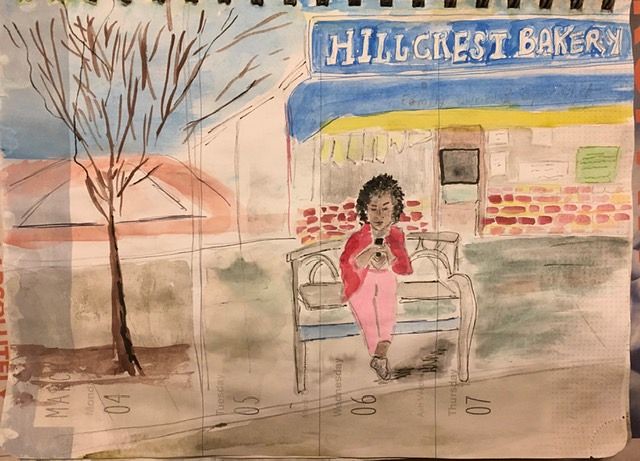This horizontal, rectangular watercolor painting captures an up-close scene of a woman sitting on a brown bench outside the Hillcrest Bakery, which features white font on a blue background. The artwork, still in its spiral-bound sketchbook, likely doubling as a calendar, adds additional contextual layers with dates like "May 4, 08, 06, 07." On the left-hand side of the image, there is a dead tree with a thin, dark brown trunk and bare branches, signifying wintertime. Behind the tree, a pink triangle with brown lines is visible, possibly another artistic element in the painting.

The woman, who has dark skin and short black hair, is dressed in a red shirt or jacket, pink pants, and black shoes. Her ankles are crossed, with her right leg over her left, and she appears engrossed in her phone, held in her hands. A brown pocketbook is situated next to her. The bakery's exterior is composed of red bricks with hints of yellow visible inside. The blue awning of the Hillcrest Bakery prominently displays the store's name in white letters. To the right of the store's door, several pieces of paper, including a green one, are tacked up, featuring black squiggly lines. The painting also incorporates mini vertical yellow rectangles hanging from a yellow beam, adding further detail to the storefront scene.

This intricate depiction, rendered on white watercolor paper, highlights both the nuanced architectural elements and the everyday moment of the woman, blending them seamlessly into the larger setting.